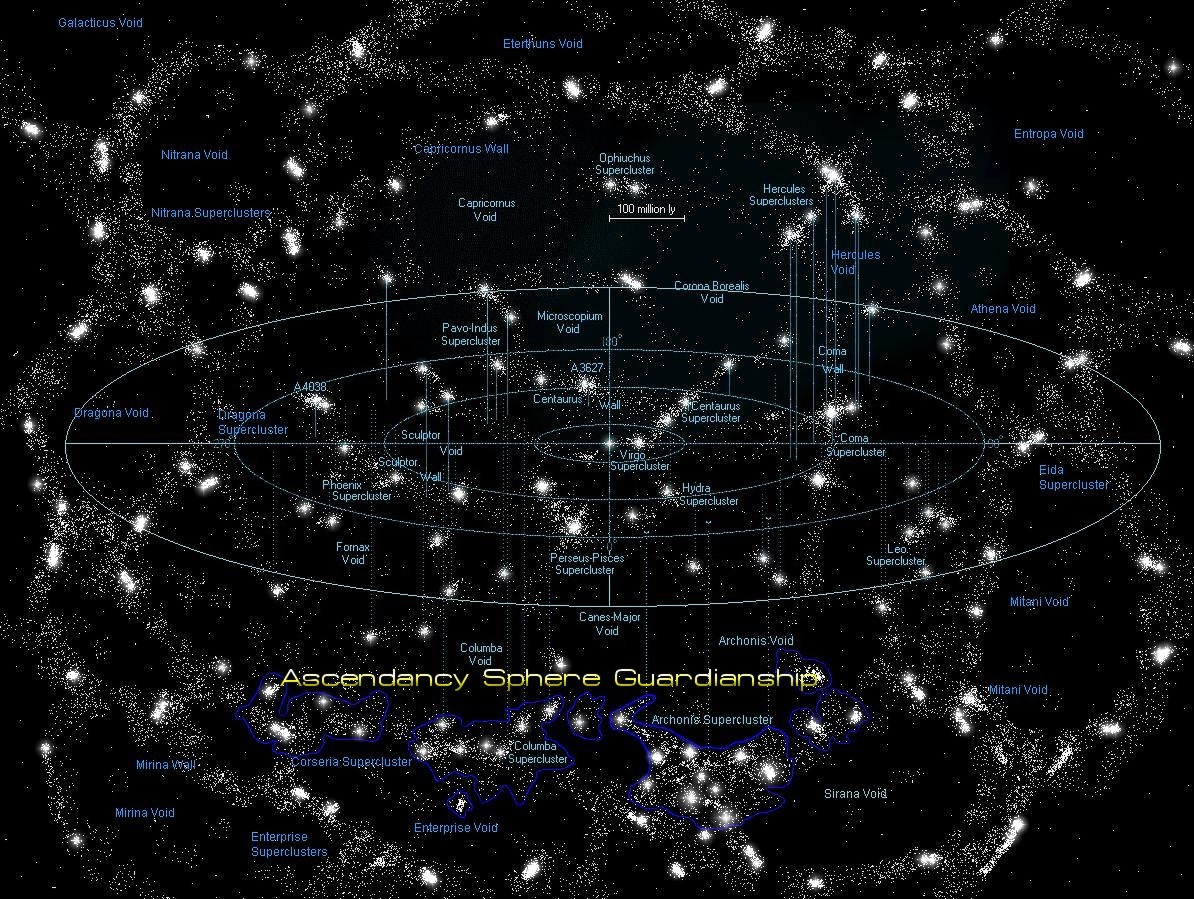The image is a horizontal rectangular depiction of a celestial map set in space. The background is pitch black, scattered with countless tiny white dots representing stars. At the center of the image are four spheres arranged in a two-dimensional plane, with three of these spheres increasing in size from the center outward. Below these spheres is a prominent inscription in yellow text reading "Ascendancy Sphere Guardianship." Surrounding these main elements, there are numerous smaller pieces of text in blue and white, labeling individual stars and celestial bodies. An axis runs through the center of the image, possibly indicating directional orientation such as north and south. The overall layout and labeling suggest this image serves an educational purpose, illustrating the arrangement and naming of stars in a specific section of the universe.